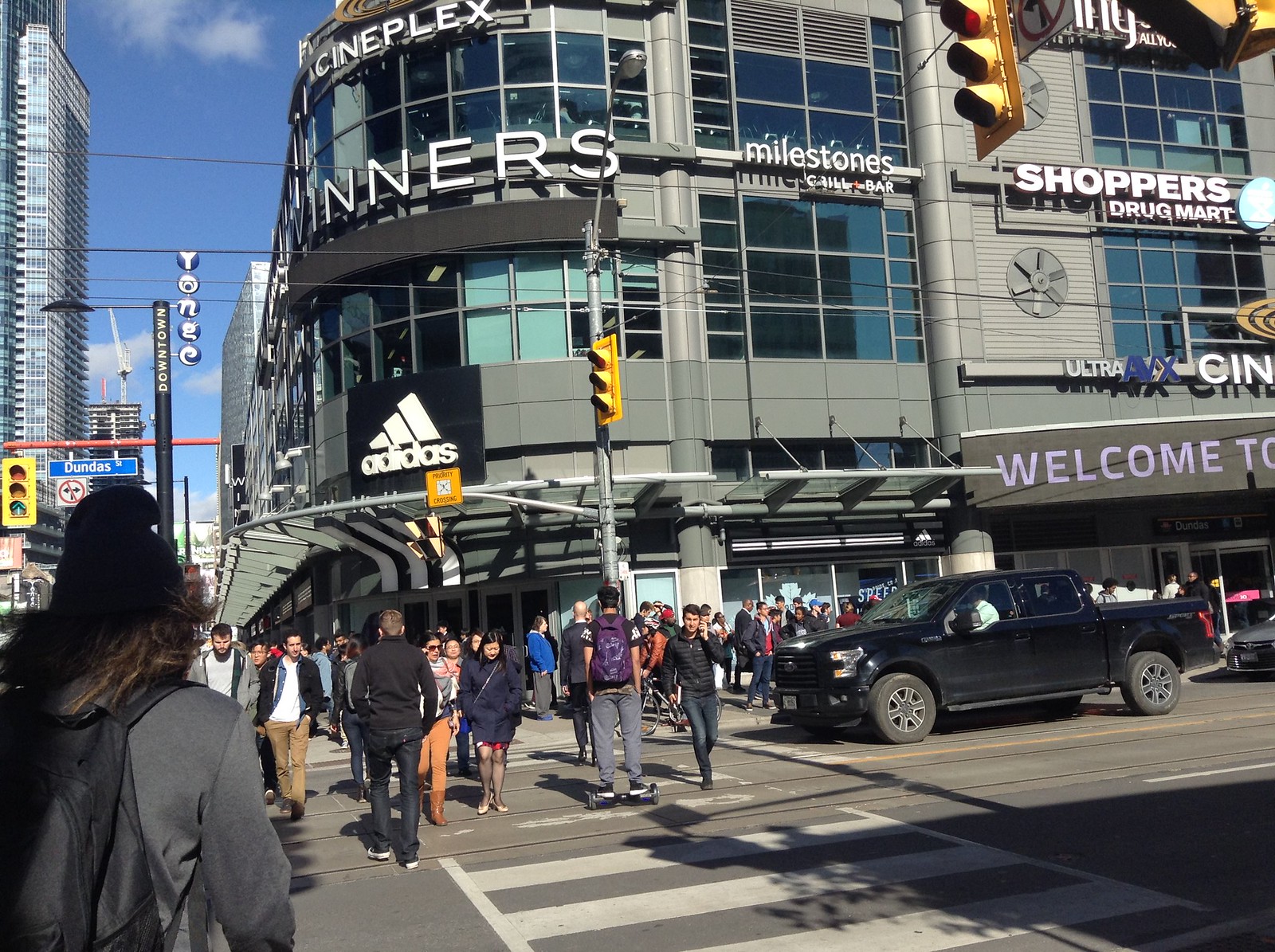This color photograph captures a bustling city street corner on a beautiful day with blue skies. The intersection is fairly busy, with many pedestrians crossing the road and walking along crowded sidewalks reminiscent of New York City. Prominently featured is a black pickup truck waiting at the light, with people walking in front of it. Taken from across the street, the image prominently shows a modern, three-story mixed-use commercial building in shades of gray. The ground floor houses an Adidas store, recognizable by its black square logo, with an overhang that wraps around the corner. Above Adidas, the storefront signage reads "Winners," and at the top of the building is a Cineplex sign, indicating a movie theater. Additional signage on the right side of the building indicates Milestones Grill & Bar and Shoppers Drug Mart. The street sign on the left reads Dundas Street, adding a sense of location to this vibrant urban scene.